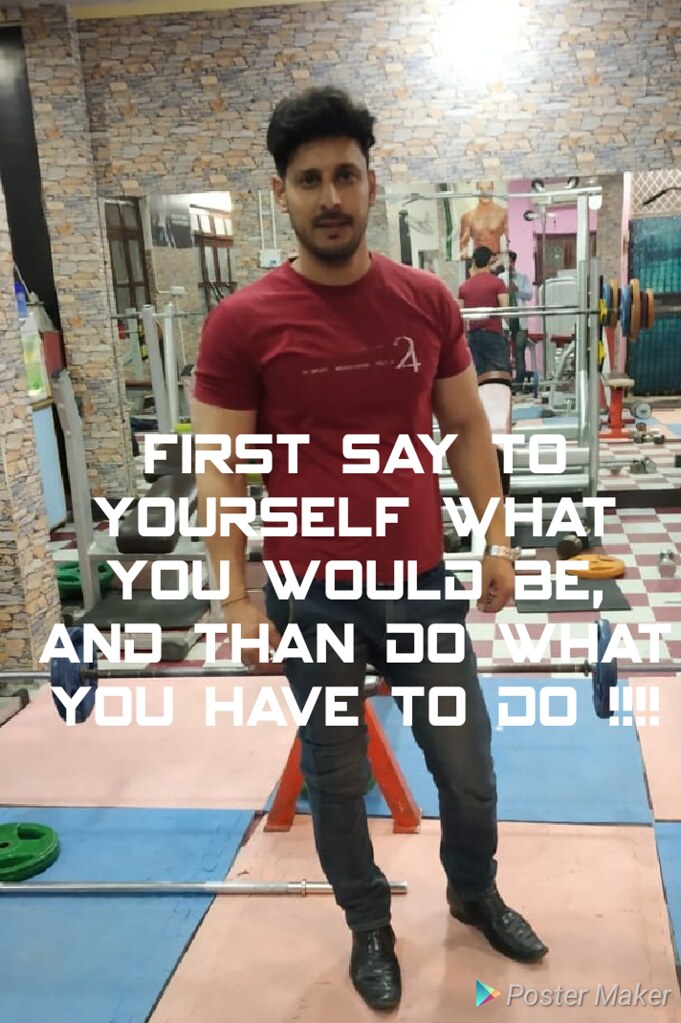In this detailed image, a young man stands in a small gym, dressed in a red t-shirt, black jeans, and black shoes. The gym floor features a pattern of alternating blue and salmon pink square mats. Surrounding him is an array of gym equipment, including an inclined bench with a barbell loaded with weights, a bar on the ground with a green plate behind him, and another barbell with blue plates further back. A mirror behind the man reflects his back and the torso of another person lifting weights. Overlaying the man in bold white text are the words, "FIRST SAY TO YOURSELF WHAT YOU WOULD BE, AND THEN DO WHAT YOU HAVE TO DO." In the bottom right corner, the name "Postmaker," accompanied by a logo resembling the Play Store, is visible. The room is dominated by stone walls, enhancing the rugged gym atmosphere.